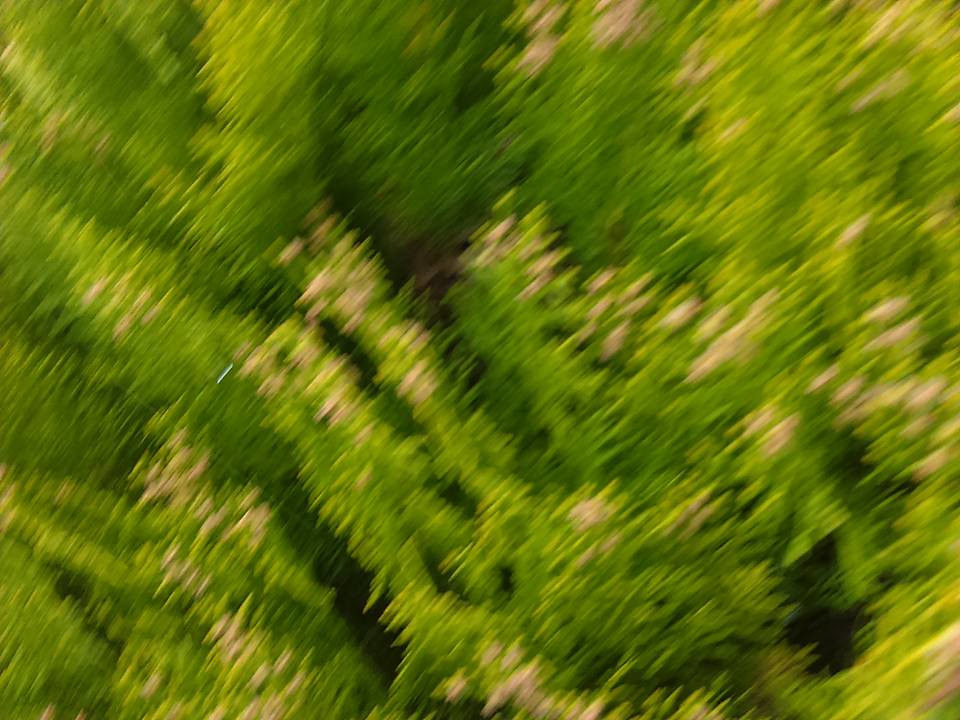This color photograph captures an aerial view of a forest, and while its dimensions are slightly wider than it is tall, the overall image is quite blurry. The greenery varies in color, presenting a gamut from dark to light greens, interspersed with patches of yellow. Amidst the foliage, there are a few darker areas suggesting gaps where trees may be sparse or missing. Despite the lack of sharpness, the image offers a faint impression of towering trees and underbrush, creating a mosaic of natural shades that hint at the lushness of the woodland below.